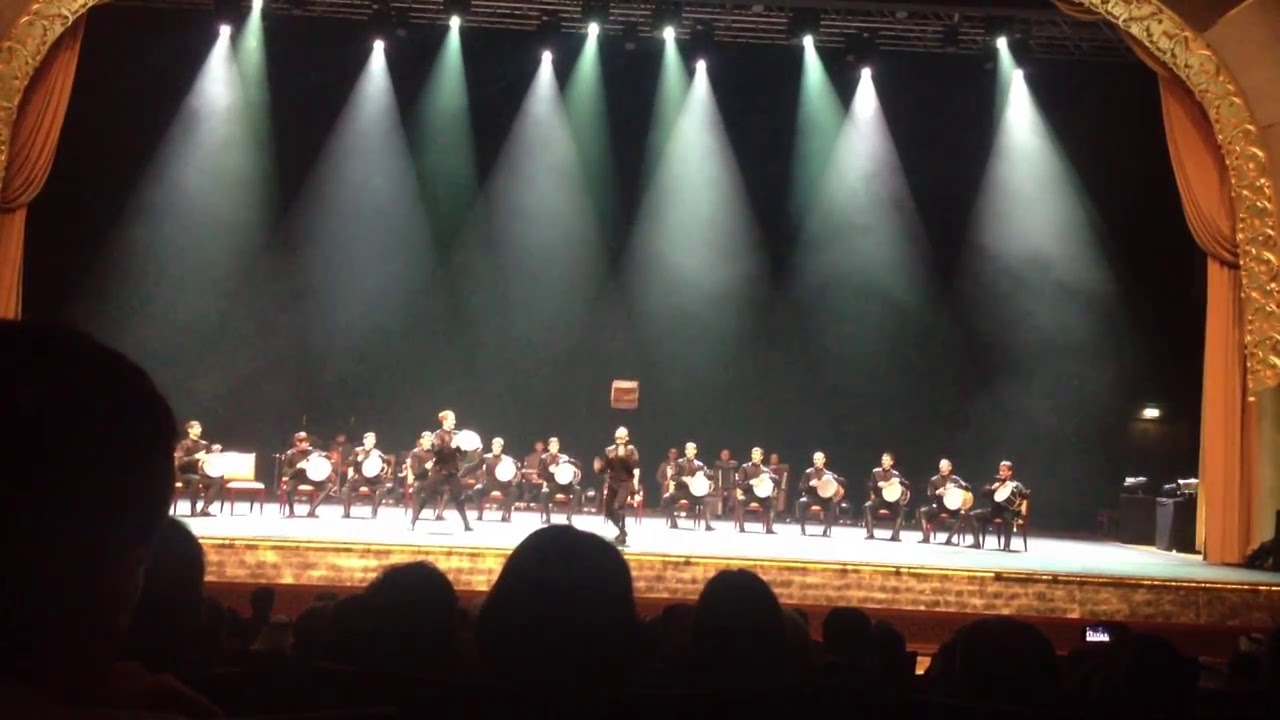The photograph captures a grand stage production set in an ornate playhouse with a vast stage framed by orange and gold ornate curtains and designs along the sides. A black backdrop enhances the dramatic lighting, with several large skylight spotlights illuminating the scene. The performers are predominantly percussionists, seated in chairs with hand drums on their laps, dressed in dark clothing that seamlessly blends with their seats. Among them stand two notable figures: one standing percussionist at the front, and another performer in the middle of an acrobatic act, balancing a box in the air, gazing intently at it. Nestled towards the back are musicians holding accordions and cellos, although they are currently not playing. The foreground reveals the audience's silhouettes, with the shadowed outlines of their heads visible. Additionally, on the lower right, someone is recording the captivating performance with their cellphone, capturing the essence of this vibrant production.